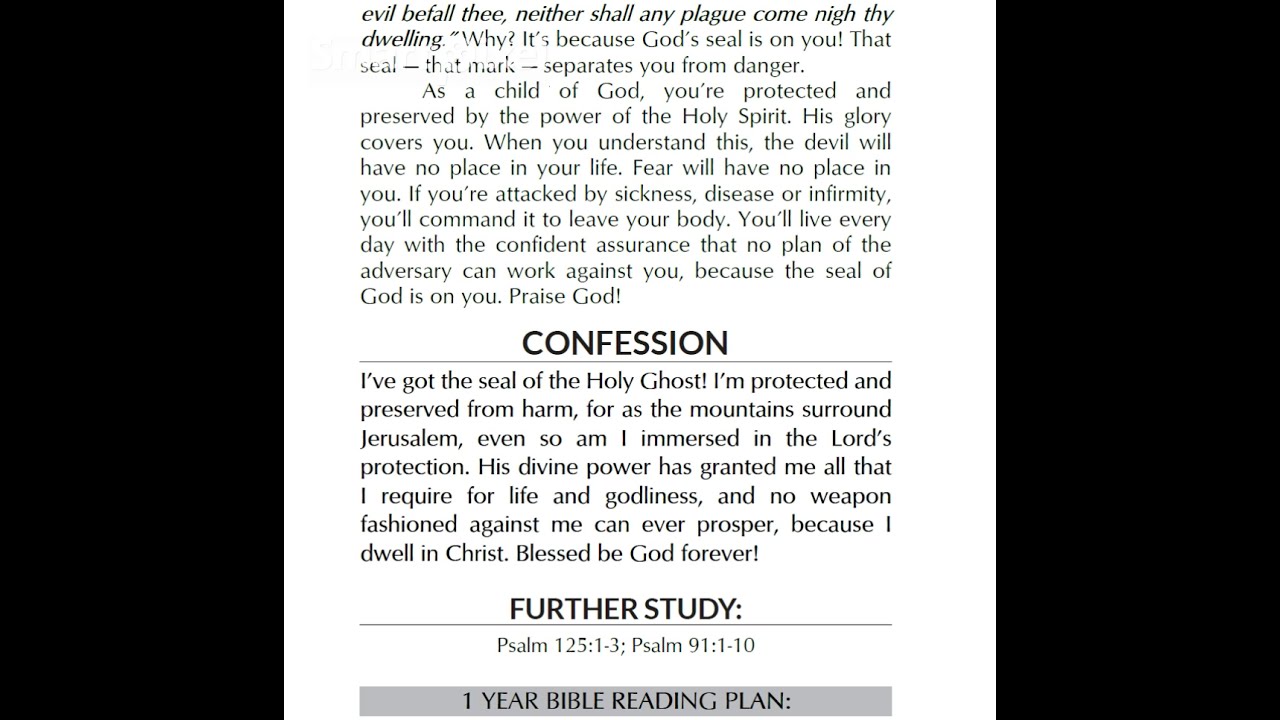The image appears to be a screenshot from a Bible study guide or religious text, with a clean, organized layout featuring a predominantly white rectangular section against a black background. The central headline, in bold and capitalized black font, reads "CONFESSION." Below this heading, there is a detailed religious affirmation stating: "I've got the seal of the Holy Ghost. I'm protected and preserved from harm, for as the mountains surround Jerusalem, even so am I immersed in the Lord's protection. His divine power has granted me all that I require for life and godliness, and no weapon fashioned against me can ever prosper, because I dwell in Christ. Blessed be God forever." This message emphasizes themes of divine protection and empowerment through faith. Beneath the main text, in capital letters, "FURTHER STUDY:" is followed by references to Bible verses Psalm 125:1-3 and Psalm 91:1-10. Below these references is another heading in black font, "One Year Bible Reading Plan," encased in a gray rectangular background. The page is visually composed with a focus on clarity and organization, containing no other objects or imagery.